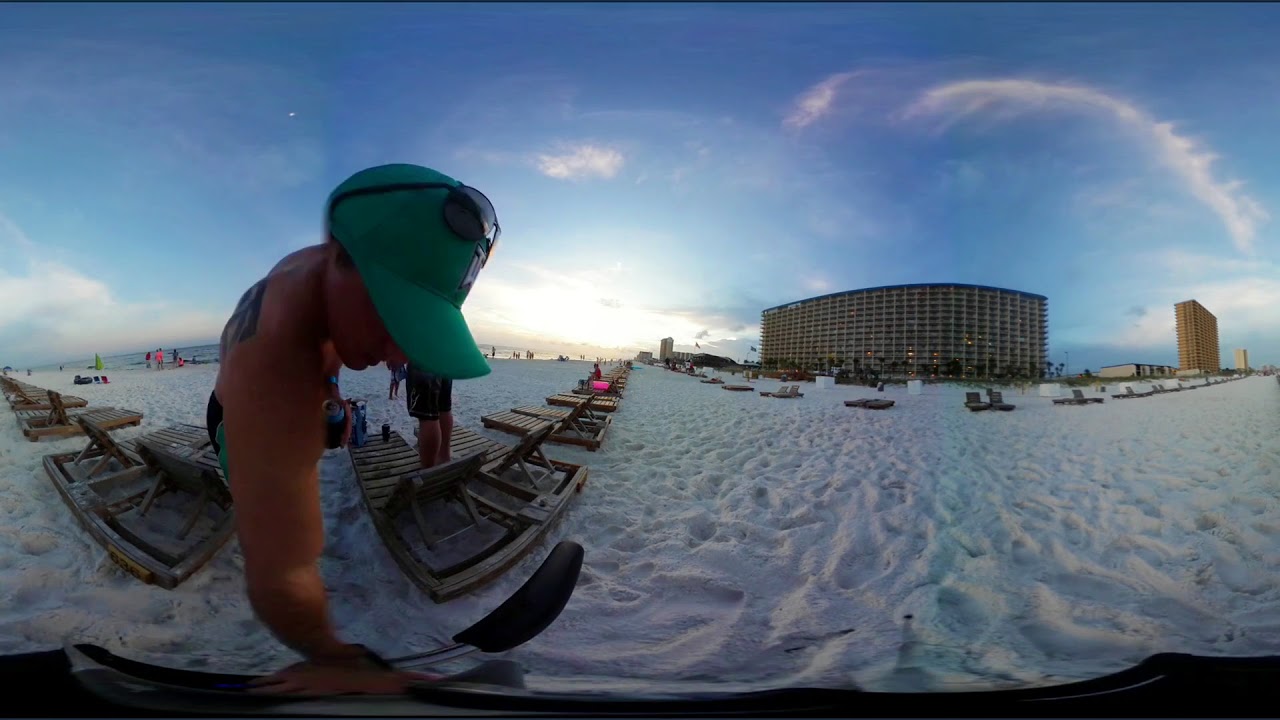A panoramic beach scene stretches across this photorealistic image, capturing the serene atmosphere of the sandy shores. The white sand, textured with numerous footprints, covers the majority of the foreground. Just left of the center, a person wearing a green baseball cap, which has sunglasses perched atop it, stands with one arm extended as if they are taking the photo. Their face is obscured as they look down, revealing a black tattoo on their exposed shoulder. This individual appears to be shirtless and dressed in swim trunks, indicating a leisurely beach day. 

Behind them, a row of wooden beach chairs extends far into the distance, curving slightly and drawing the eye toward the horizon. Adjacent to these chairs and closer to the ocean, you can see more people gathered near the water, which is visible on the left-hand side behind the person. 

In the background, on the right side of the image, stands a multi-story building, brown in color and difficult to detail from this distance, which resembles a large hotel or condominium. More structures are visible further left, including additional beach chairs that are closer to the water. The sun sits low in the bright blue sky, suggesting either morning or evening, and is accompanied by wispy clouds, enhancing the tranquil, picturesque setting.